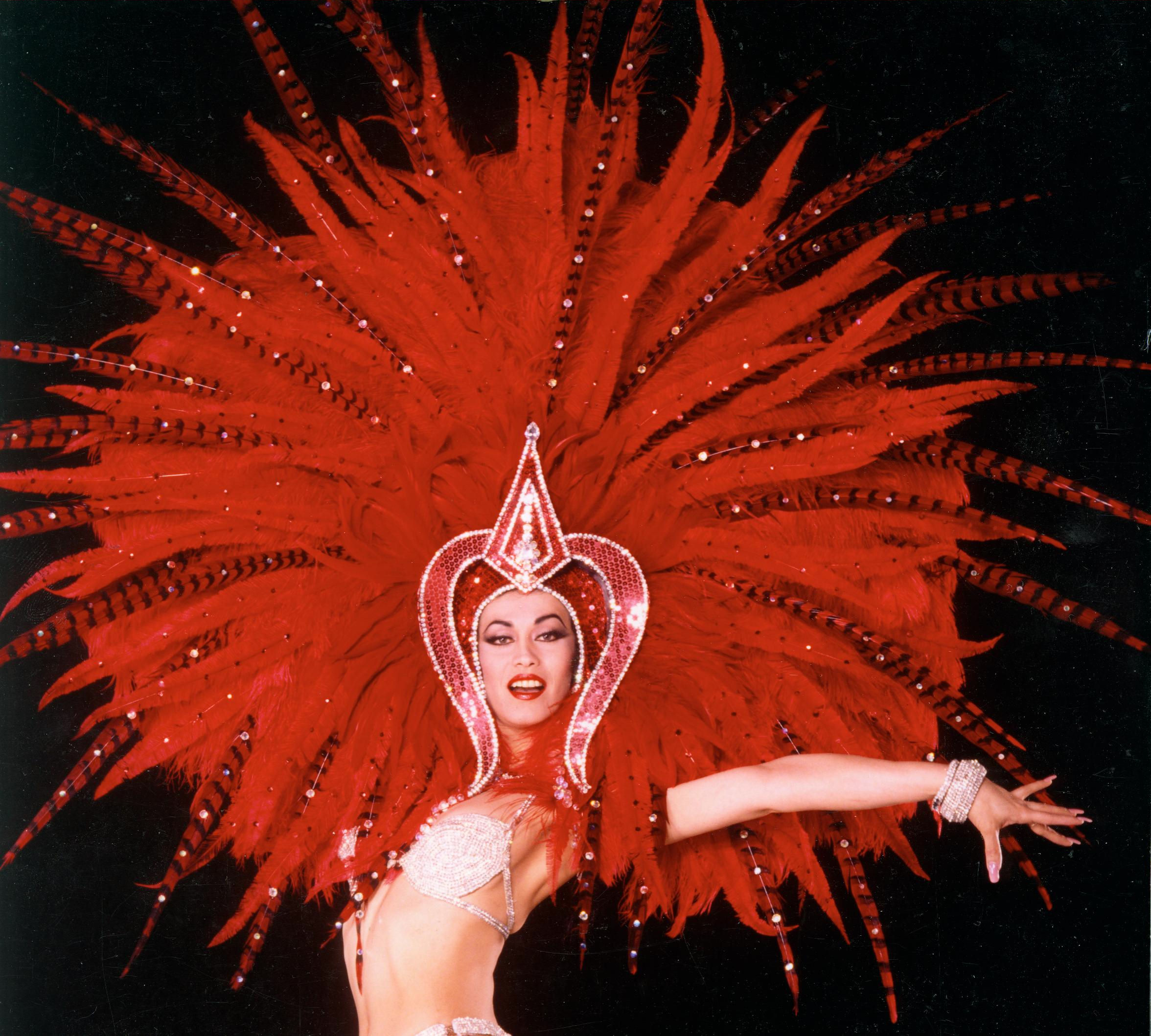The image depicts a vintage photograph of a showgirl, likely from a Las Vegas revue. The background is solid black, bringing sharp focus to the glamorous figure from her waist upward. She wears a jewel-encrusted, silver bikini top, and the image offers a glimpse of her similarly ornate bottom at the lower edge. Her face is adorned with bright red lipstick and meticulous makeup, her mouth slightly open to reveal her upper teeth. The headdress she dons is a spectacle unto itself, a massive, flamboyant display of red feathers interspersed with black-striped feathers laden with gems, fanning out extensively and extending beyond the frame. This elaborate headdress features a central, gem-studded triangular design with side elements that resemble poofy waves framing her face. She poses with her body turned to the left while her left arm extends elegantly to the right, showcasing a thick, sparkling diamond-like bracelet and her long, splayed fingernails. The image captures the essence of showbiz extravagance in every detail.